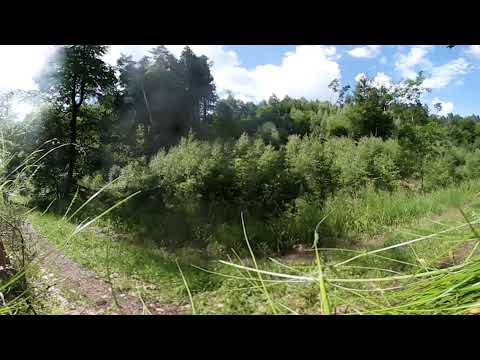The photograph depicts an outdoor scene that looks like a lush forest or dense woods, featuring an abundance of greenery. The main focal point is a dirt path, visible on the left side of the image, marked by the faint tracks of a car, hinting that it might rarely be used; it isn't a well-defined road as weeds and grass encroach upon it. This path is surrounded by a rich tapestry of nature, with various shades of green from grass, bushes, shrubs, and different species of trees. The background showcases taller trees, while the middle ground highlights medium-sized bushes, complemented by shorter grass in the foreground, including some almost yellowish-green patches to the bottom right. The sky is partly visible, painted with blue and dotted by fluffy white clouds, indicating a sunny and pleasant day. The scene is devoid of any animals, people, or text, presenting an untouched and serene natural landscape.